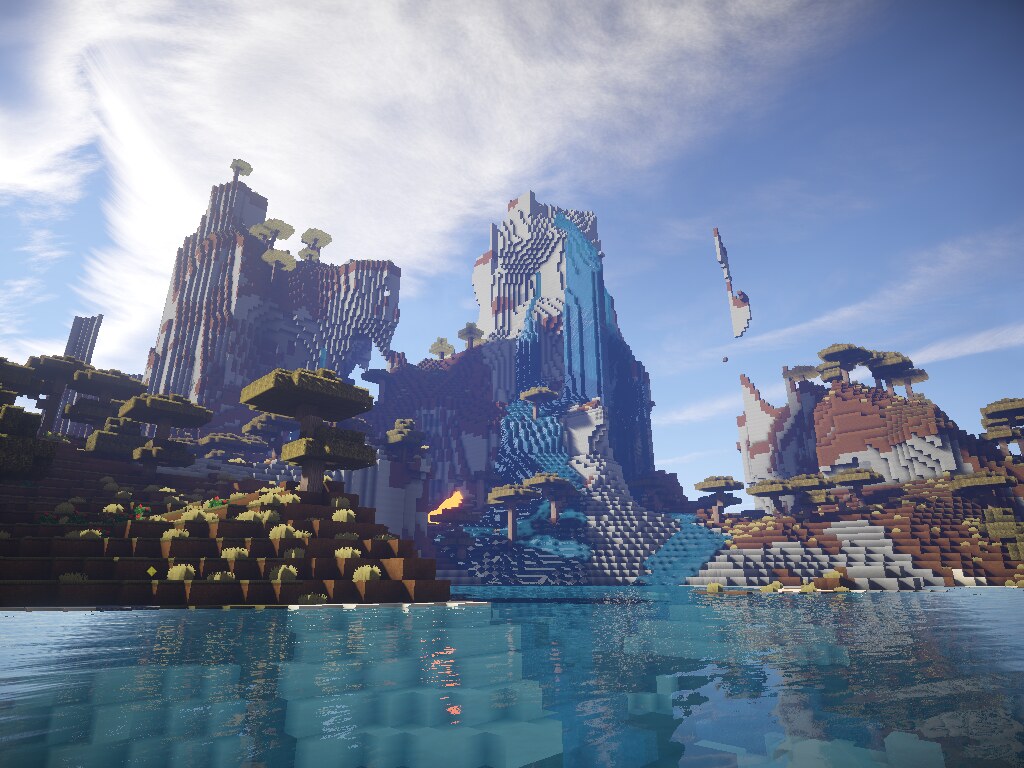The image is a vibrant, computer-generated landscape reminiscent of Minecraft, featuring various structures made entirely of pixelated, block-like elements. In the foreground, a turquoise blue body of water stretches across, mirroring the fantastical environment around it and revealing a submerged terrain composed of similar pixel blocks. The left side showcases a brown blocky bank topped with yellow tufts resembling grasses or weeds.

Prominently, the background is dominated by three towering, block-constructed mountains. These mountains, crafted from a mix of white and brown cubes, look snow-capped and covered with sparse trees made of green blocks, with the left mountain hosting six visible block-trees. A blue sky filled with scattered, wispy clouds emphasizes the surreal ambiance.

Several structures in the scene introduce a sense of architectural whimsy, diverging from standard shapes to include pillars and possibly a central building with notable blue sections. The landscape creates an imagined, fantasy world constructed with a digital tool reliant on block mechanics, invoking the aesthetics of games like Minecraft.